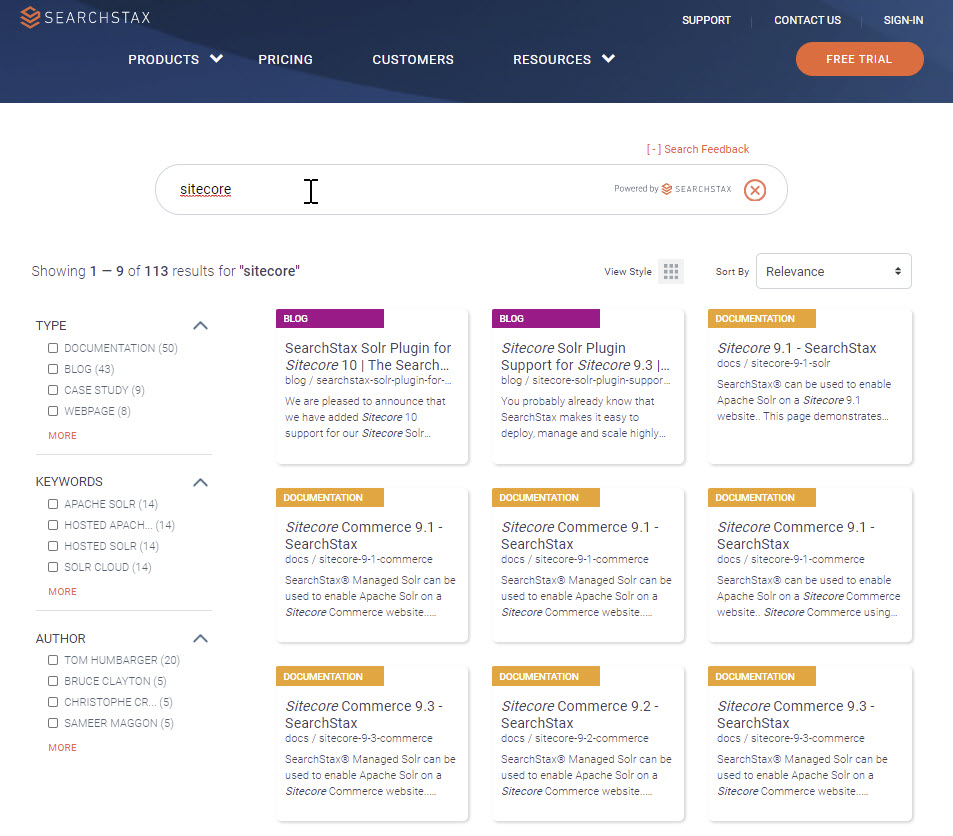This image is a screenshot of a website interface. In the upper left-hand corner, the text "Search Stacks" is prominently displayed. On the upper right-hand side, there are navigation links labeled "Support," "Contact Us," and "Sign In."

Beneath this top section, aligned towards the left, there are four clickable buttons labeled "Products," "Pricing," "Customers," and "Resources." On the right-hand side of this row, there is a button marked "Free Trial."

Below this navigation bar, a search bar is prominently featured. The term "SiteCore" has been entered into the search field, and on the far right end of the search bar, the text "Powered by Search Stacks" is visible.

Directly beneath this search bar, towards the left-hand side, the caption "Showing 1 to 9 of 113 results for SiteCore" is displayed. Along the left-hand side of the page, filtering options are available. 

The first filtering section is labeled "Type" and includes options to filter by "Documentation," "Blog," "Case Study," "Webpage," and more. The second section, titled "Keywords," lists filters such as "page," "Solar," "hosted page," "hosted Solar," "Solar Cloud," and additional options. 

The final filtering section is labeled "Author," listing names like Tom Humberger, Bruce Clayton, Christopher (the last name is cut off), and Samir Magin.

This detailed screenshot showcases a user-friendly search interface with multiple filtering options to narrow down search results.